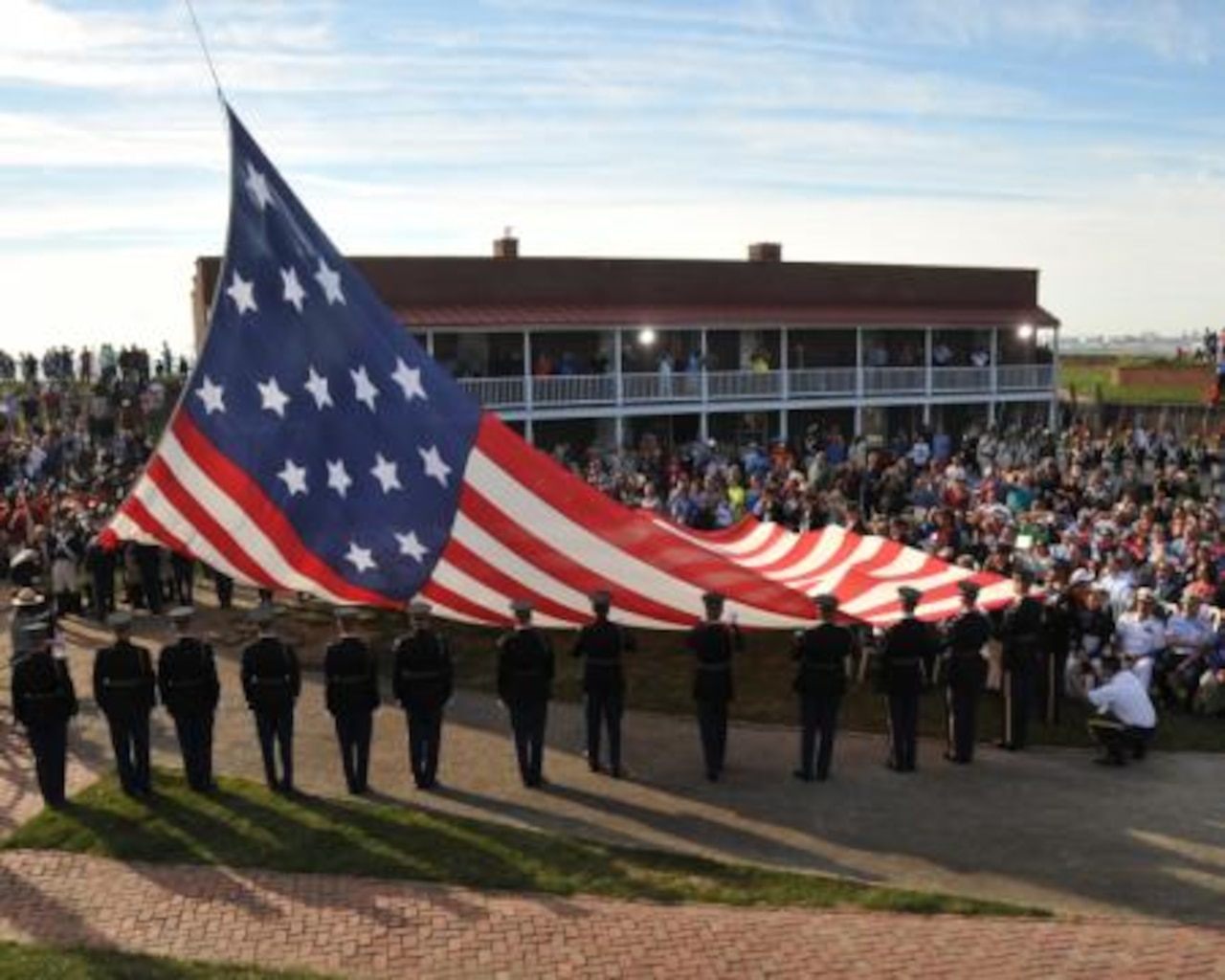This photograph captures a military ceremony taking place outdoors, likely at the start or end of an event. Centered in the image is a massive American flag, showcasing its red, white, and blue colors with white stars in a blue square. The flag is being held or prepared to be raised by a line of military officers, distinguished by their dark blue uniforms adorned with yellow stripes down the sides and dark blue hats. Surrounding the ceremony is a large, engaged audience, with some people standing on the upper deck of a nearby two-story building, holding onto the railing and possibly taking pictures. The scene is slightly blurry, indicating motion and activity, and the lighting suggests it is either early morning or late afternoon. The entire scene exudes a solemn yet celebratory atmosphere, highlighted by the large gathering of onlookers and the impressive display of military precision and patriotism.